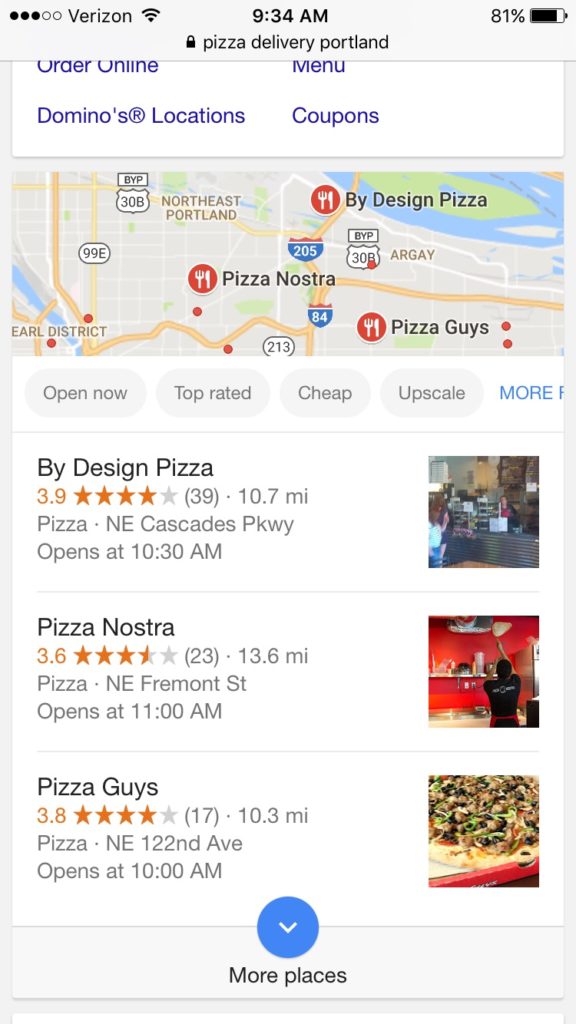The image is a screenshot from an iPhone displaying Google Maps search results for "Pizza Delivery Portland." The status bar shows the time as 9:34 AM, with a Verizon cellular signal at 3 out of 5 bars, a full Wi-Fi signal, and the battery at 81%. Below the search query "Pizza Delivery Portland," the interface provides options to "Order Online," view the "Menu," check "Domino Locations," and explore "Coupons."

The map showcases various pizza places in the Portland area marked with red dots and icons of a fork and knife, indicating they are restaurants. Below the map, filtering options such as "Open Now," "Top Rated," "Cheap," and "Upscale" are available but not selected.

Three pizza places are highlighted:

1. **By Design Pizza**
   - Rating: 3.9 stars
   - Reviews: 39
   - Distance: 10.7 miles away
   - Opening Time: 10:30 AM

2. **Pizza Nostra**
   - Rating: 3.6 stars
   - Reviews: 23
   - Distance: 13.6 miles away
   - Opening Time: 11:00 AM

3. **Pizza Guys**
   - Rating: 3.8 stars
   - Reviews: 17
   - Distance: 10.3 miles away
   - Opening Time: 10:00 AM

Each listing is accompanied by a thumbnail image to the right of the restaurant's name.